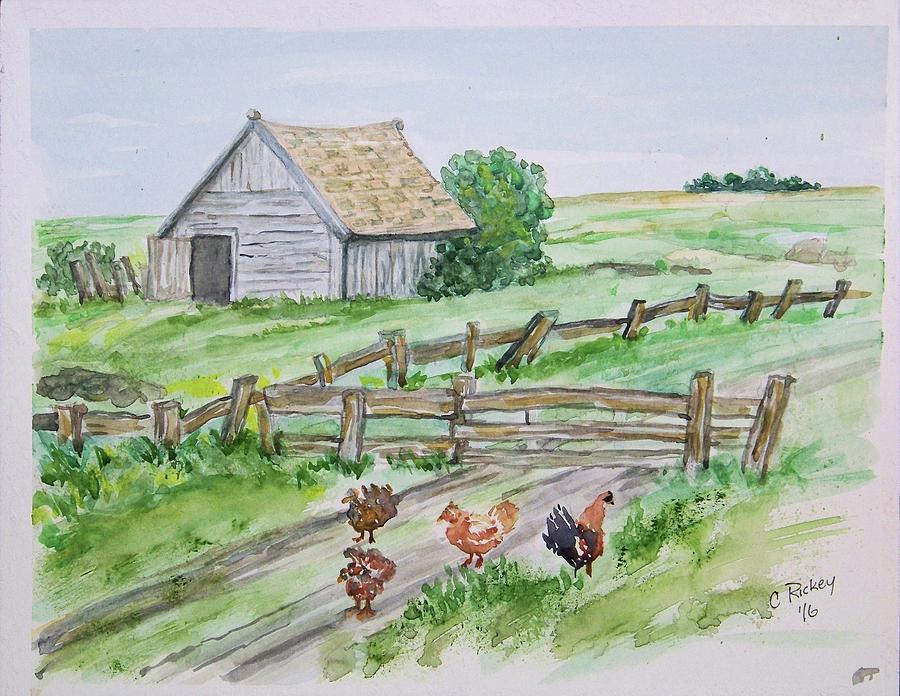The image captures a photograph of a rectangular watercolor painting with a white border, done on a white canvas or paper. In landscape orientation, the artwork predominantly features a serene farm scene. The upper third of the painting displays a light blue sky with streaks of white clouds. Below, there is a gentle, rolling green hill adorned with small shrubs and trees. Prominently situated towards the top left is a wooden barn or shed with a light brown roof. To the right of the barn stands a solitary tree. 

A fence, intersecting at a right angle, runs horizontally from the barn, creating a partition in the landscape. A worn-down trail for a vehicle cuts through, moving from the bottom left corner towards the center right, where it meets the fences. Scattered along the trail are four chickens, including what appears to be one rooster. The painting is signed in black in the bottom right corner with the artist's mark, "Sea Ricky 1/6."